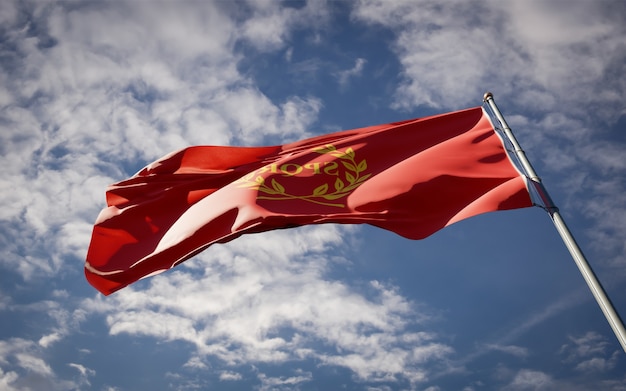This photograph captures a vivid scene of a red flag prominently displayed against a backdrop of a clear blue sky dotted with wispy, mid-level white clouds. The viewpoint appears to be from the ground, looking upwards at the flagpole, which is a shade of gray. The flag is highlighted by bright sunlight, causing it to cast soft shadows and sunspots due to its gentle flutter in the moderate breeze. The red flag features a yellow logo in its center, composed of the letters "S-P-O-R" in large, capitalized yellow font. Surrounding the text is a circular pattern resembling a wreath, made of two stems with leaves. The flag extends from the middle right of the photo, angling slightly towards the left, anchored to the pole by a couple of visible strings. Only the upper part of the flagpole is visible as it stretches from the lower right-hand corner, emphasizing the upward perspective of this daytime shot.